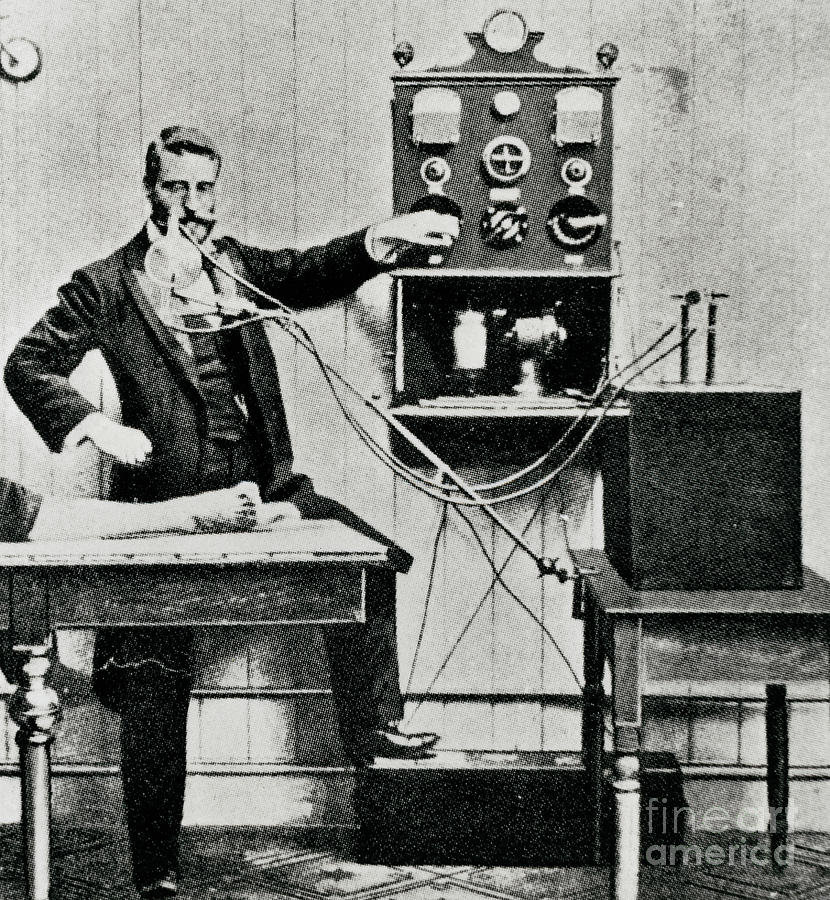This is an early black-and-white or sepia-toned photograph, likely capturing a moment from the late 19th or early 20th century, something reminiscent of Alexander Graham Bell’s era. In the bottom right corner of the photograph, the words "Fine Art America" are visible. The image features a man who could be Alexander Graham Bell, identifiable by his black hair and beard, standing in front of a wooden wall. He appears to be involved in an experiment with a complex device that includes a cylinder with tubings connected to a black box on a nearby table. The man is dressed in a long black jacket and black pants, with his left leg propped up on a black case, exposing his foot. His left hand is touching part of the equipment, suggesting interaction with a telephone machine or another early communication device. A microphone on a long arm stands in front of him, and assorted instruments and wires are scattered around, adding to the scientific aura of the scene. Off to the left, an examination table is also partially visible. The overall setting evokes a sense of historical technological experimentation.